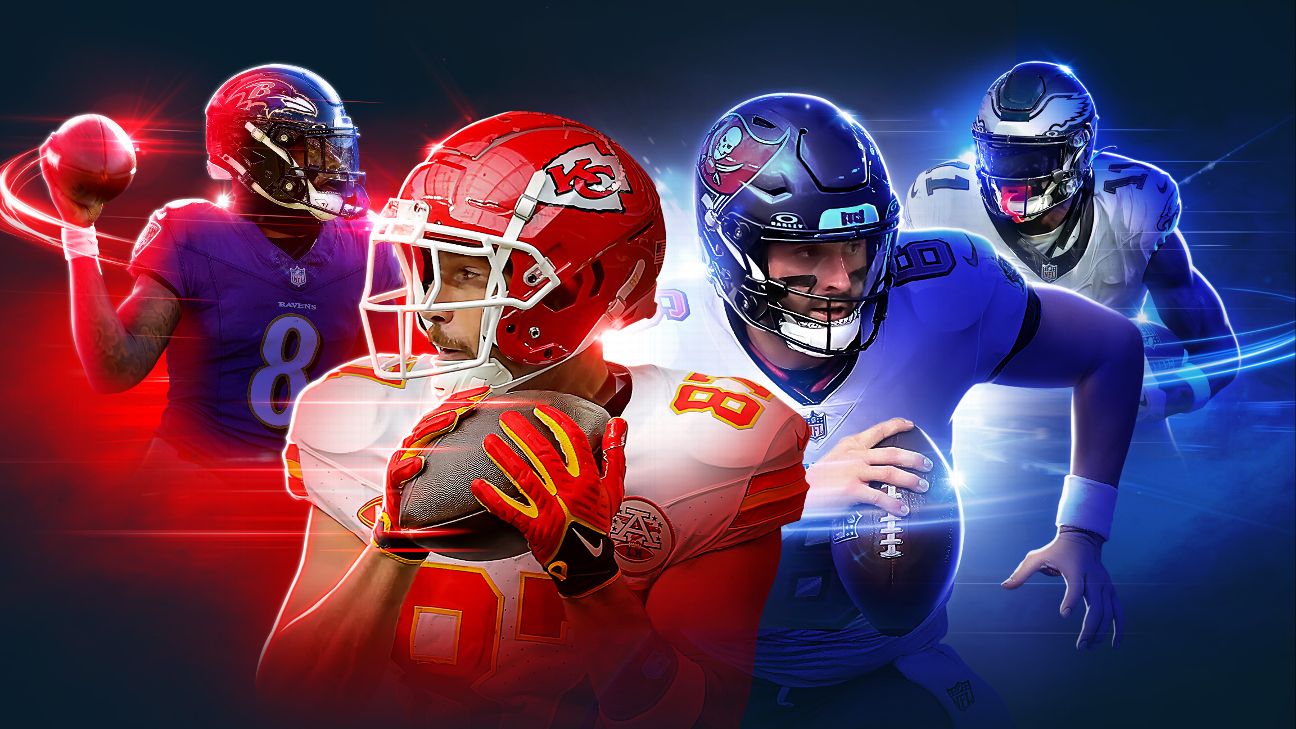This image is a highly stylized and digitally enhanced collage of four NFL football players. On the left, an Afro-American player from the Baltimore Ravens, distinguishable by his helmet with a bird logo, is poised to pass the football. Next to him, in the foreground, is a Kansas City Chiefs player, number 81, wearing a red helmet and white jersey, holding the football with both hands and looking to his left. Third from the left is a player from the Tampa Bay Buccaneers, wearing a white jersey and dark helmet, captured mid-run with the football in his right hand. The player all the way on the right, possibly from the Philadelphia Eagles, has Apollo's wings on his helmet, and he is bathed in an electric blue light. The two players on the right are distinguished by blue neon lighting, while those on the left are illuminated with red light, enhancing the vivid and futuristic atmosphere of the image. All players are depicted in action poses, with helmets and face masks in place, set against a vignetted background that emphasizes their dynamic and energetic stances.